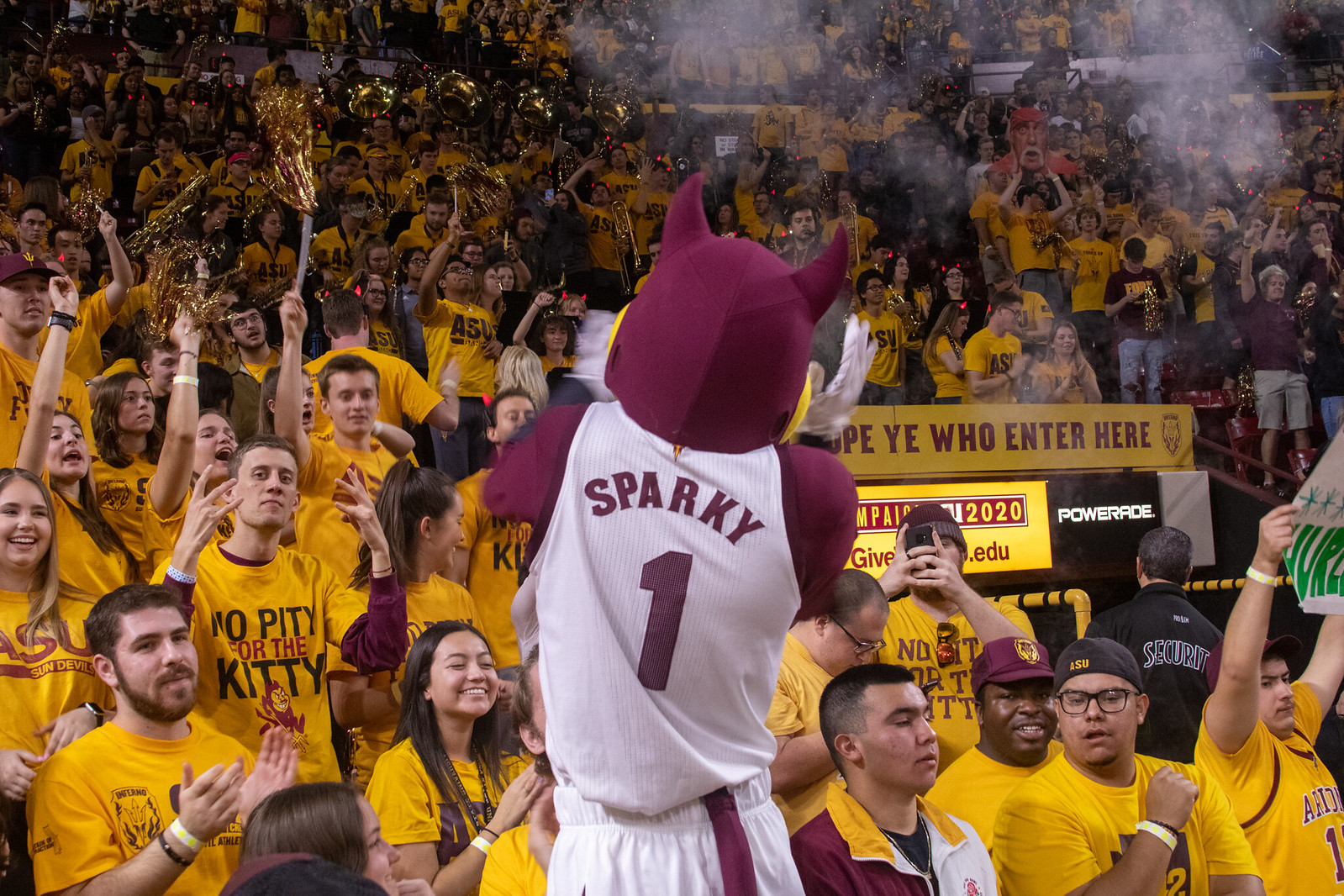The image captures the vibrant atmosphere of a college football game at Arizona State University, showcasing the lively crowd of fans in the stands. The stands are filled with college-age students, most of them clad in yellow t-shirts, embodying the school spirit with sparklers and pom-poms. Front and center in the image stands the ASU mascot, Sparky. Sparky, depicted as a maroon devil-like creature with horns and bird-like features, dons a white basketball jersey marked with "Sparky #1" and white trousers. A visible hat in the front row features the letters "ASU," further suggesting the location.

The crowd's energy is palpable, with many fans smiling and one even capturing the moment with a camera. Another fan's t-shirt reads "No Pity for the Kitty," featuring an image of Sparky. There's a mixture of smoke in the air, possibly from a nearby kitchen. In the background, the higher rows reveal a section of the school's band, with trombones and gleaming tubas contributing to the festive atmosphere. A sign above an entrance or exit in the seating area reads "Abandon all hope, ye who enter here" alongside a partially obscured advertisement, possibly for a 2020 campaign. The full energy and spirit of game day at Sun Devil Stadium are beautifully encapsulated in this snapshot.